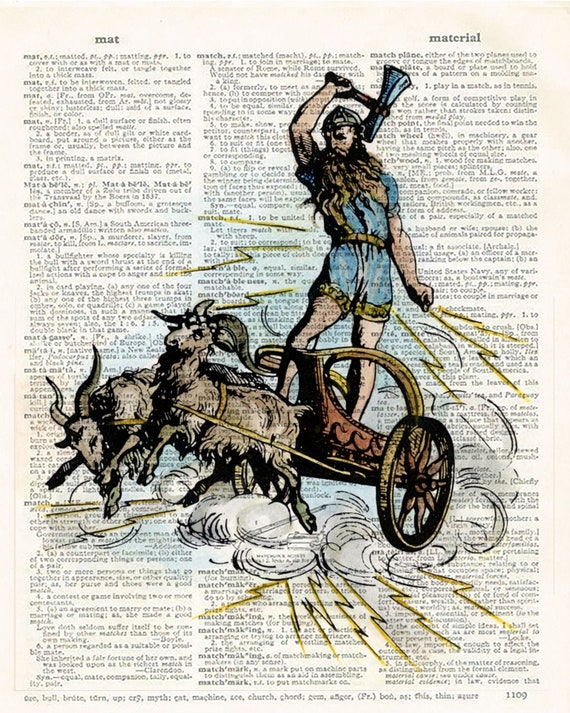This illustration, drawn over an off-white, yellowed dictionary page featuring the words from "mat" to "material" in three columns, depicts an ancient warrior in vivid detail. The warrior, with a long flowing brown and blonde beard almost reaching his waist, wears a blue, short-sleeved onesie adorned with gold trim around the waist and thighs. He stands firmly in a small, two-wheeled wooden chariot, drawn by two struggling goats with exceptionally long horns. The man, his full front facing the viewer, wields a short-handled axe or hammer high over his head, as if ready to strike. The artwork includes straight-line yellow lightning bolts radiating from his body and the chariot’s frame, adding a mythical, possibly divine element to the scene, suggesting the warrior's immense power. The page’s text, though minuscule and not intended to be read, forms a backdrop that highlights the dynamic and vibrant central illustration.